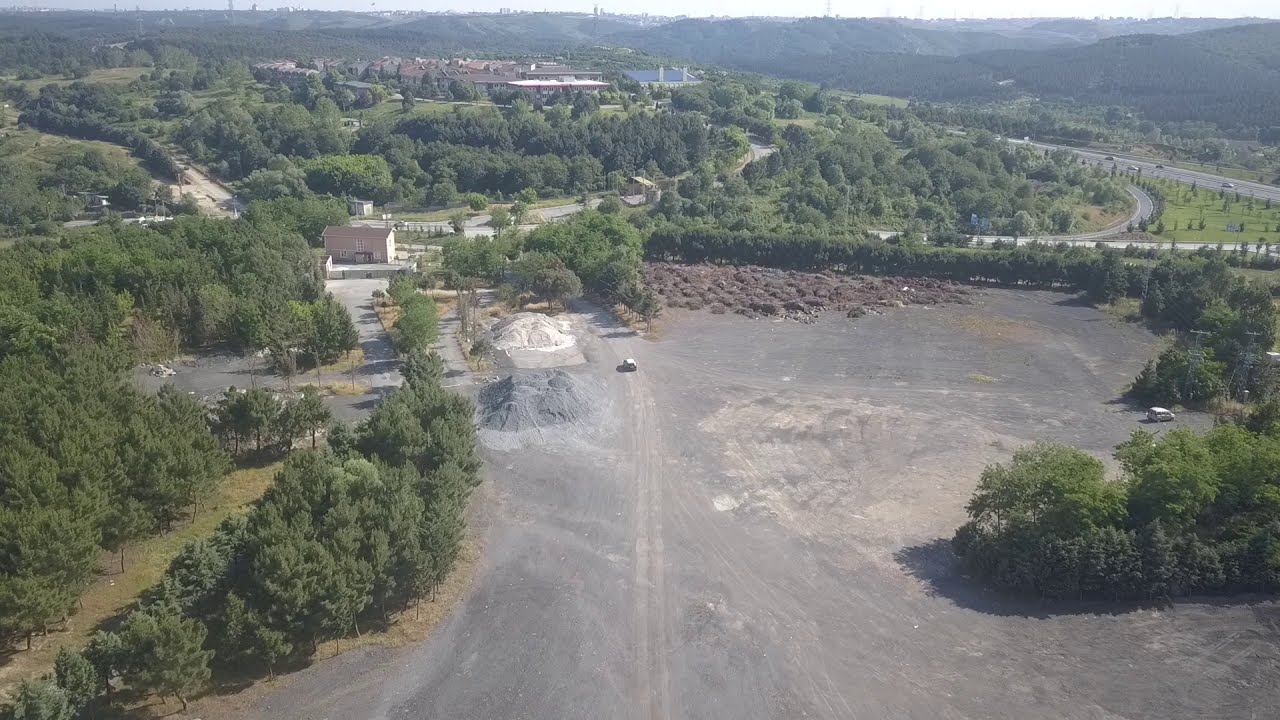This aerial view captures a diverse landscape transitioning from a large industrial lot in the foreground to a verdant neighborhood stretching into the distance. The foreground features a sprawling gravel and dirt space, dotted with various dump loads, possibly bark chip from a mill, sawdust, and piles of gravel. This industrial area is traversed by a dirt road with a car navigating through it. Surrounding this open lot are thick clusters of lush green trees and bushes.

Moving beyond this industrial zone, the scenery shifts to a vibrant neighborhood. This residential area, characterized by a mix of homes and commercial properties, is crisscrossed by streets lined with more dense greenery. In the distance, the neighborhood expands into a subdivision with additional homes nestled against a backdrop of green hills, some of which have exposed patches of dirt.

To the right of the neighborhood, a highway runs adjacent to a forested area, where a road winds through the dense canopy of trees towards a central city area with buildings. The verdant landscape continues up to the foothills of encompassing green mountains, under a white sky that looms above, infusing the scene with a sense of vastness and continuity.